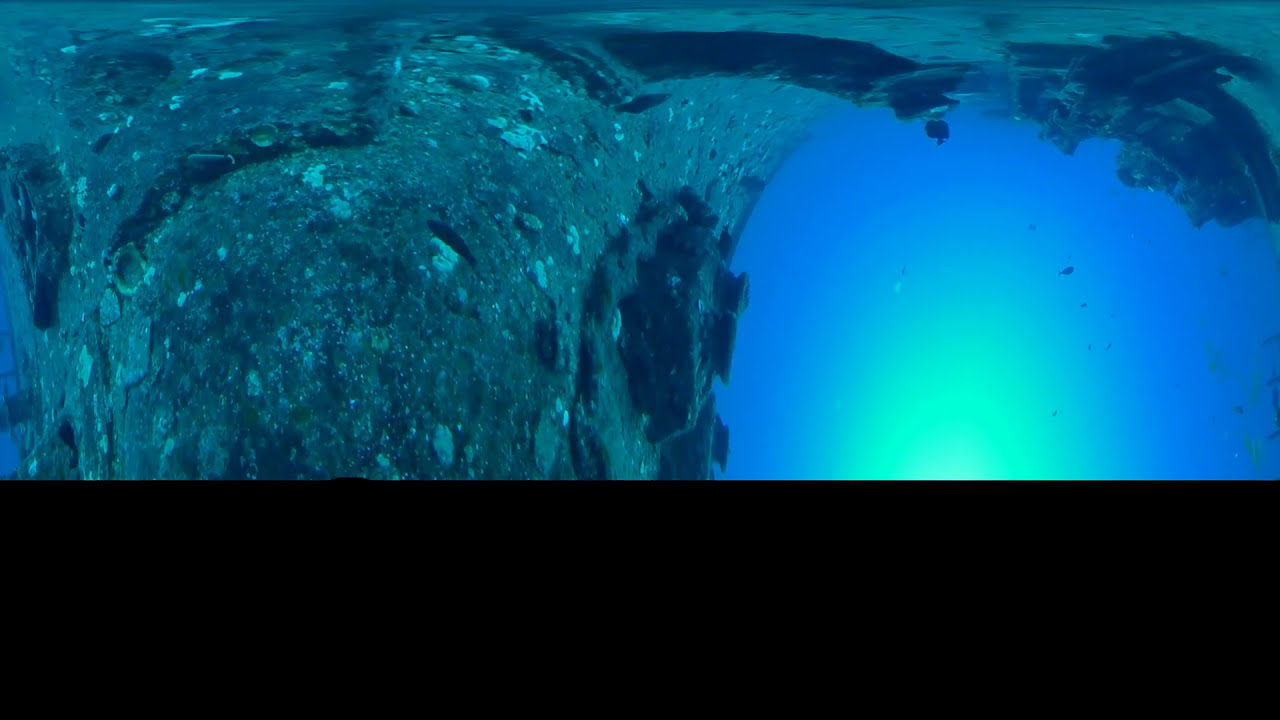This image, likely taken underwater, captures a scene with a strong perspective that makes it appear as if it is tilted or inverted. Dominating the lower section is a thick, black border that occupies about one-third of the image. On the top and extending towards the left, there is a large, textured stone area or possibly the ocean floor, featuring various pebbles and intricate details, including light and dark patches, shells, and black rocks. The stone structure curves upwards with somewhat warped edges, giving the impression of depth and an underwater landscape.

In contrast, the bottom right corner of the image reveals clear, open water with light blue and dark blue hues, and possibly a few indistinct fish swimming about. From this vantage, the surface of the water reflects sunlight, casting a blue-green tint around the top right, adding to the underwater ambiance. Despite the image's distortion, the setting clearly depicts an outdoor underwater environment, bathed in daylight, without any visible text. The color palette ranges from black and shades of blue to gray, white, and tan, contributing to the natural, aquatic feel of the scene.